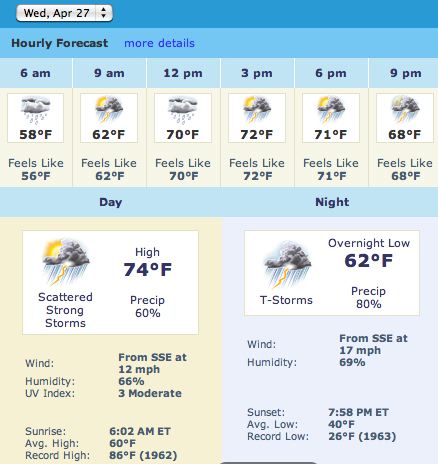The image depicts an hourly weather forecast for Wednesday, April 27th. At the top, navigation arrows allow for date selection, flanked by the headings "Hourly Forecast" and "More Details." The forecast spans from 6 a.m. to 9 p.m.

- At 6 a.m., it is 58°F and raining, feeling like 56°F.
- At 9 a.m., it will be partly sunny at 62°F, feeling like 62°F.
- By 12 p.m., it will rain with a temperature of 70°F, feeling like 70°F.
- At 3 p.m., expect thunderstorms and partly cloudy skies at 72°F, feeling like 72°F.
- At 6 p.m., it will be partly sunny with thunderstorms, at 71°F, feeling like 71°F.
- At 9 p.m., thunderstorms are forecasted with a temperature of 68°F, feeling like 68°F.

Below the hourly forecast, a banner divides the day and night details. For the day:

- There will be scattered strong storms with a high of 74°F.
- Precipitation chance is 60%.
- Winds will come from the south-southeast at 12 mph.
- Humidity will be at 66% with a UV index rated 3 (moderate).
- Sunrise is at 6:00 a.m. Eastern.
- The average high is 60°F, while the record high was 86°F in 1962.

For the night:

- The overnight low is 62°F with thunderstorms.
- Precipitation chance rises to 80%.
- Winds continue from the south-southeast at 17 mph.
- Humidity increases to 69%.
- Sunset is at 7:58 p.m. Eastern.
- The average low is 40°F, while the record low was 26°F in 1963.

Images accompany the forecast, illustrating the expected weather conditions, such as suns for sunny intervals and storm clouds for thunderstorms.